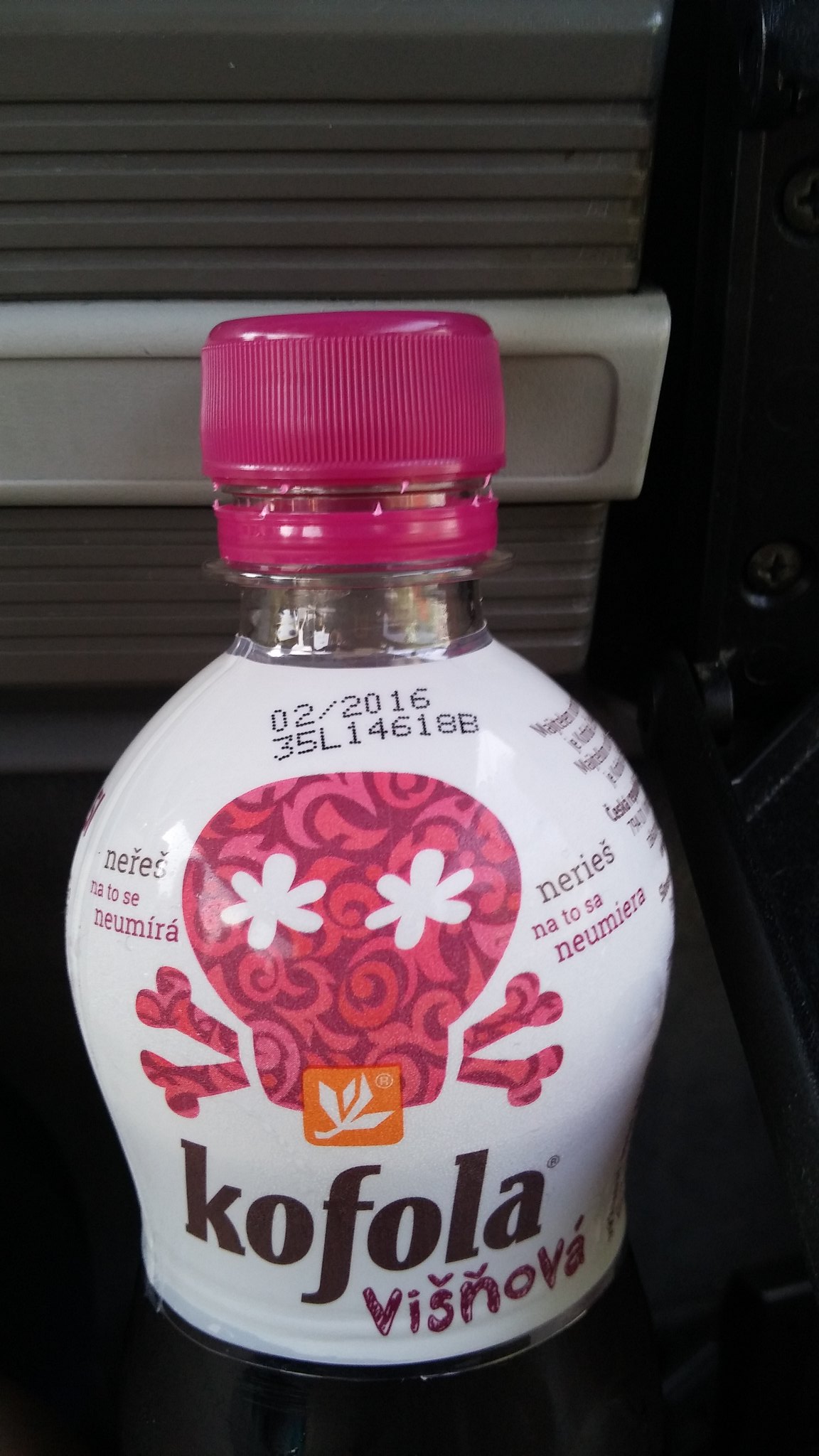This detailed close-up image captures a short, squat plastic bottle with a pinkish-purple screw cap and cap ring, set against a grey backdrop on a black counter. The bottle's bulb-like body is primarily white, adorned with an intricate label. Central to the label is a pink skull with crossbones, characterized by various shades of pink and white flower-shaped eye sockets. Notably, there is an orange square with a white leaf in the mouth area of the skull. Below this motif, the text "Kofala Viznova" stands out, with "Kofala" in a dark font and "Viznova" in a mauve or pinkish hue. Additional writing is present along the sides of the label. Near the neck of the bottle, stamped on the white part, is the date "02-2016," likely indicating an expiration date.